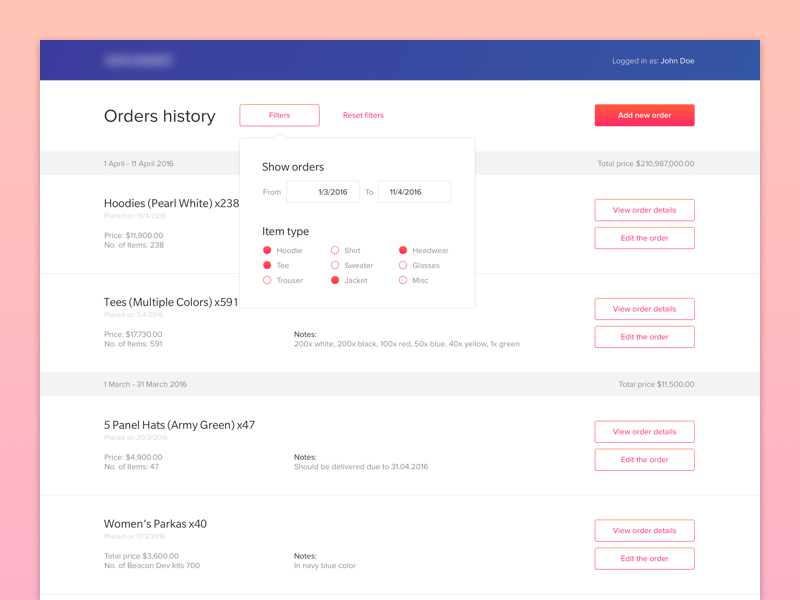Here's a detailed and cleaned-up caption for the image:

"The window features an ombre background transitioning from a light peach color at the top to a pastel hot pink color at the bottom. At the top right, a dark violet header displays small white text that reads 'Logged in as:' followed by 'John Doe' in a brighter white. On the left side, there is additional white text that is blurred out. Below, the window shifts to a white background with 'Orders History' written in black at the top left and 'Filters' to the right. The word 'Filters' is encased in a hot pink rectangular shape with a pink-filled center.

Beneath this, there is a dropdown menu with a square, light gray border and 'Show orders' written in black. Two boxes for date selection are positioned to the left, labeled 'From' in light gray. The first box contains '01/03/2016' in black, followed by 'to' in gray, and the second box displays '11/04/2016' in black. Below this section, 'Item Type' is written in black on the left, listing several radio button options.

The radio options are highlighted in hot pink when selected. 'Hoodie' and 'Tee' are selected, indicated by the filled-in circles. 'Trouser' is presented with an unselected hot pink bordered circle. On the next row, 'Shirt' and 'Sweater' are also unselected. 'Jacket' has a dark pink filled circle, indicating it is selected. On the following row, 'Headwear' is selected with a dark pink filled circle. The remaining options, 'Glasses' and 'MISC' (Miscellaneous), are unselected with hot pink bordered circles."